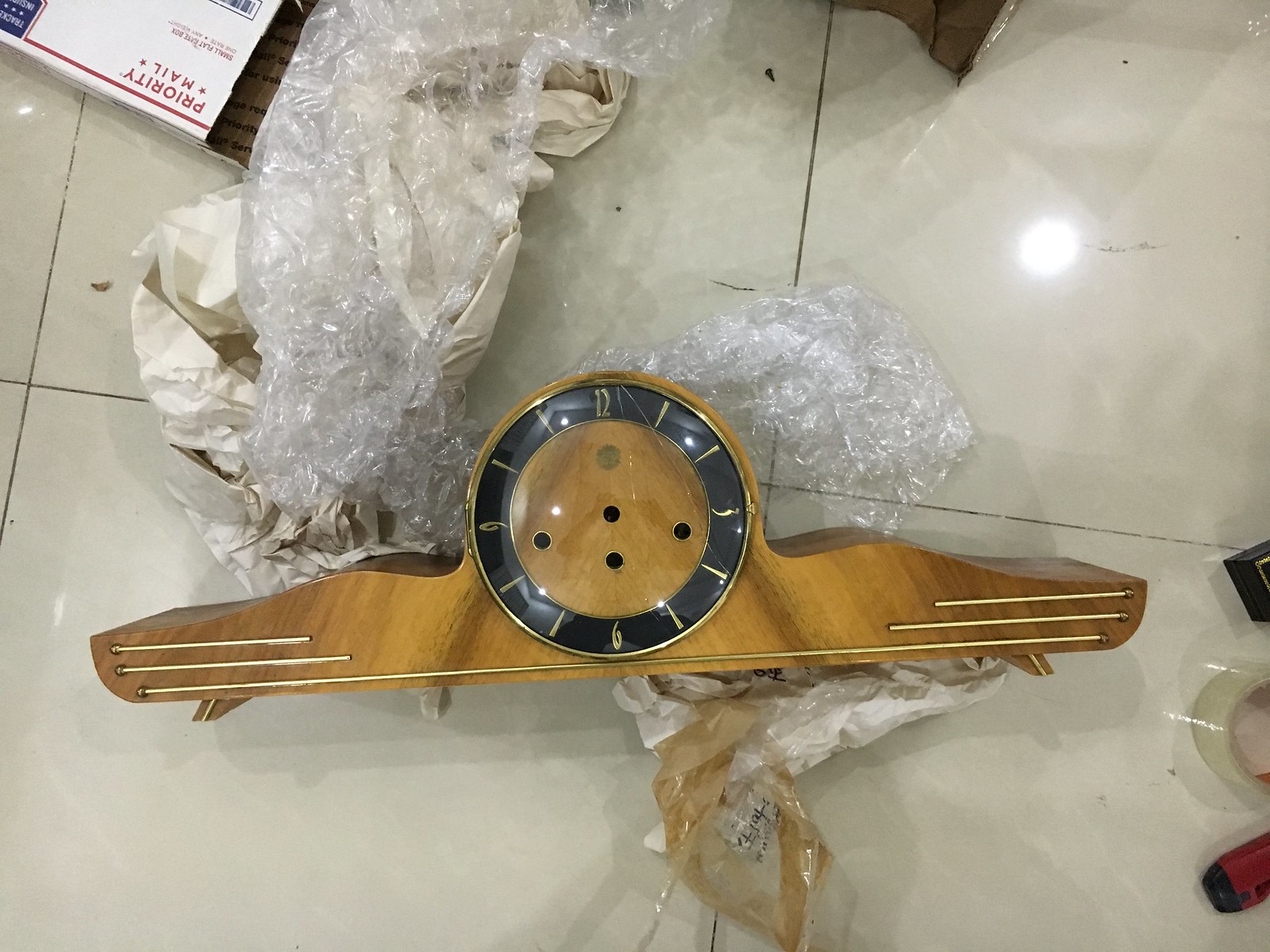A close-up photograph captures a vintage clock, noticeably worn from age and missing its protective front glass, which lies shattered. The clock, seemingly from the 1920s based on its distinctive numerical fonts and design, features a wooden structure with a round central face flanked by wing-like extensions on either side. It is placed atop a layer of bubble wrap and paper, suggesting recent shipping. In the upper left corner of the frame, a "Priority Mail" box reinforces the idea of its shipment. The entire scene is set against a backdrop of white tiled flooring, highlighting the antique clock's intricate design and current state of disrepair.